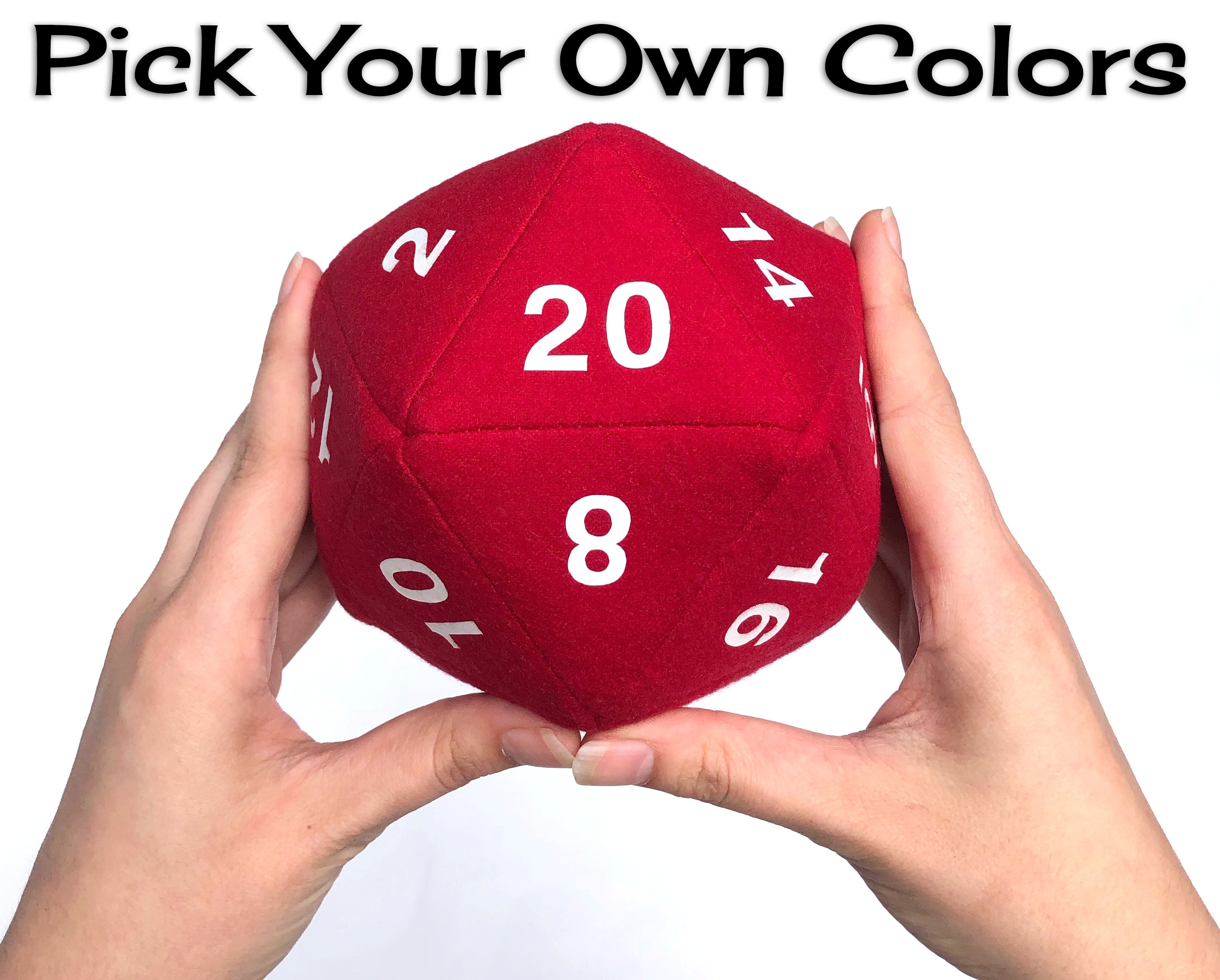The image features a pair of human hands holding a plush, jumbo-sized 20-sided die, vividly colored in bright red. The plush die, which resembles a dodecahedron, is composed of triangular surfaces, each emblazoned with a white number. The triangular faces visible show the numbers: 20 on the top central face, flanked by 2 (upper left), 14 (upper right), 8 (lower central), 10 (lower left), and 16 (lower right). The hands are positioned such that the thumbs meet at the base of the die, while the fingers grip its sides. The backdrop is a clean white, and across the top of the image, printed in bold black letters, is the text "Pick Your Own Colors."